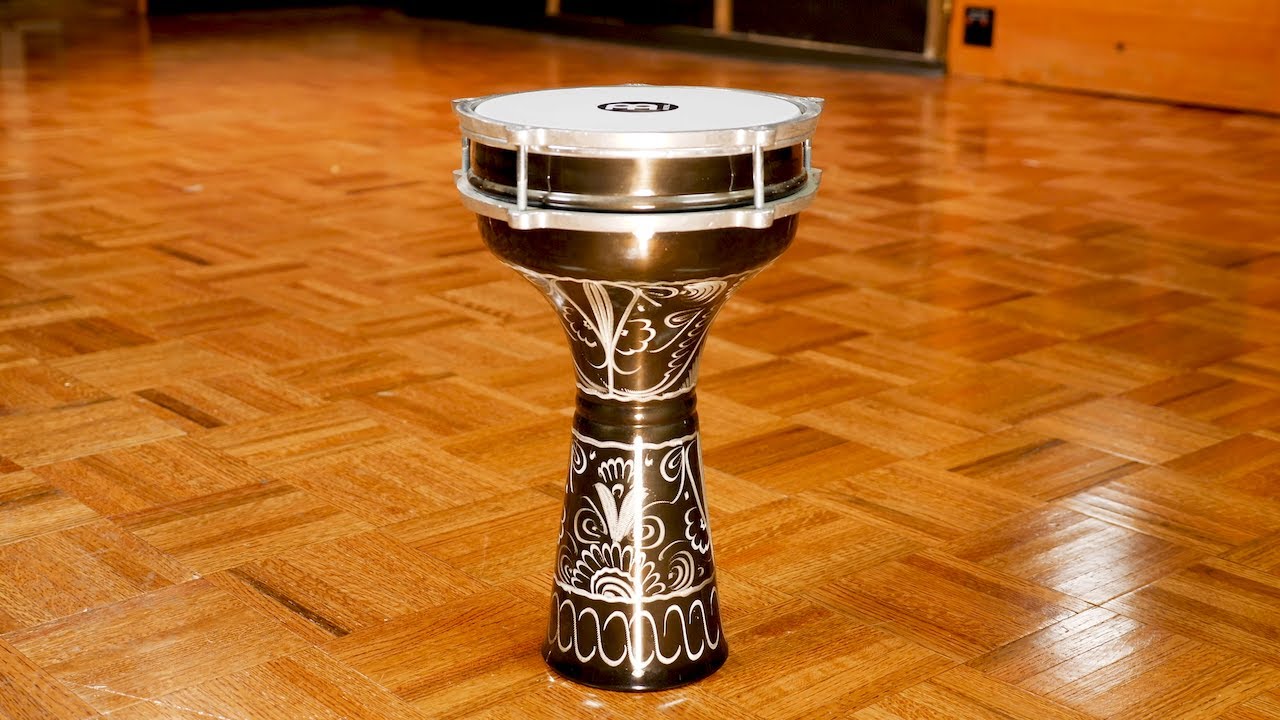The photograph features a beautifully decorated drum with a metallic coppery and white finish, intricately adorned with hand-drawn white designs that include swirly patterns, mandalas, and floral motifs. The drum has an hourglass shape that rises from a circular base on the floor to waist height, culminating in a drum surface that is white with a prominent black circle in the center. This striking object is placed alone in the middle of an expansive, glossy parquet floor comprised of small, alternating squares, indicative of an older building style. In the background, the bottom part of a glass door, a segment of a wall, and an electrical outlet are visible, slightly contrasting with the drum’s artisanal elegance.